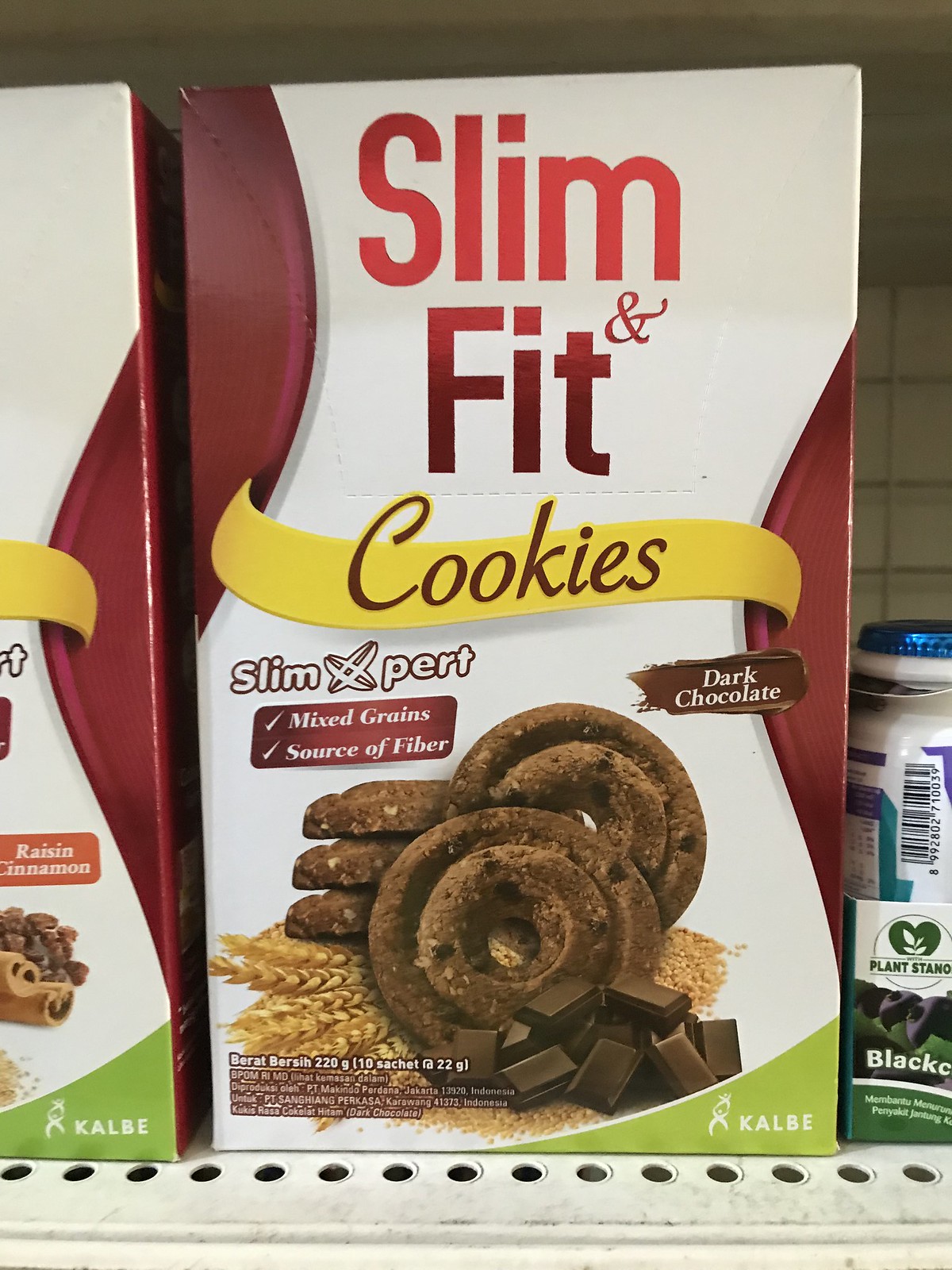The image depicts a grocery store shelf with a prominent package of Slim and Fit cookies. The main box is predominantly white with red trim and a fading red logo at the top that reads "Slim & Fit." Across the middle of the box is a yellow ribbon banner with the word "cookies" written in brown. To the right, on a dark chocolate smear, "dark chocolate" is written in white. Below the banner, a red section lists "Slim Pert," and beneath it, two check-marked claims in white text: "Mixed Grains" and "Source of Fiber." Dominating the bottom half of the box is an image of the cookies, which are circular with two concentric rings and a central hole, positioned on stalks of wheat and surrounded by bits of dark chocolate. The bottom right corner of the package features the brand name "KALBE" and a stick-figure logo. Nutritional information, including "220 grams" and "10 sachets, 22 grams each," is also present. Flanking the Slim and Fit cookies are another box of Slim and Fit cookies, partially cut off on the left, and a bottle of what appears to be plant-based milk with a metallic blue cap and a blue and green label to the right.